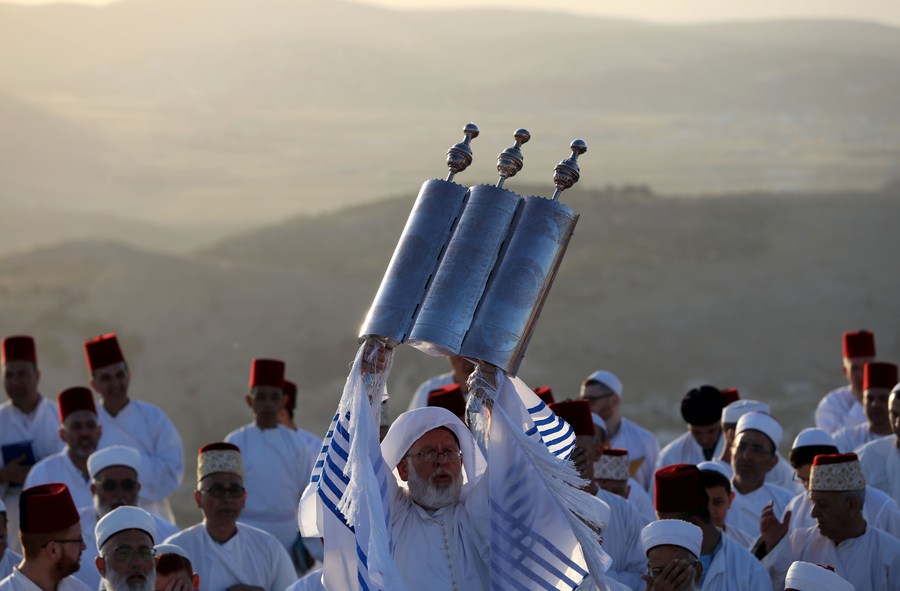The photograph depicts a group of men standing outdoors against a somewhat blurred background. The upper part of the image is dominated by a light gray sky and indistinct mountain ranges or land. Lower in the image, the landscape shifts to darker tones suggestive of a more solid terrain. The focus, however, is on the group of men garbed in white robes. Some wear white caps, while others sport deep maroon, velvet-like hats reminiscent of a Shriner's fez, adorned with a distinctive pattern.

In the foreground, prominently positioned in the center, is an older man with a thick white beard and mustache. He wears a white robe accented by a scarf-like garment with blue stripes draped over his shoulders and arms. His head is covered with a white cloth. He also wears glasses. This man holds aloft a striking, decorative object comprised of three interconnected silver cylindrical shapes, each topped with a small knob. The cylindrical tubes are linked together, and the formation gives the impression of ceremonial or religious significance. The other men in the image direct their gaze towards this central figure, emphasizing the importance of the moment.